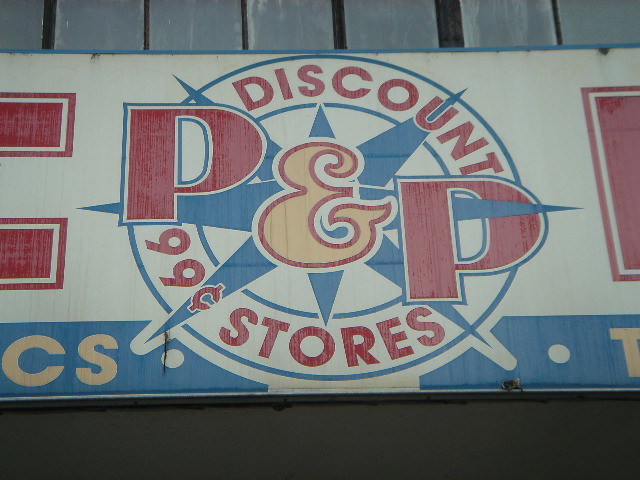A store sign for "Discount P&P 99 Cent Stores" prominently features red text against a white background. The ampersand symbol is colored yellow, adding a pop of contrast. There's a blue star in the background, contributing to the sign's vibrant appearance. Along the bottom of the sign, a blue stripe provides additional visual interest. The sign appears to be mounted on a gray or wooden siding, likely above a storefront, suggesting it's positioned to attract customers outside the store. The zoomed-in image focuses on the bold red text, white backdrop, and blue accents, making these colors the most noticeable elements.